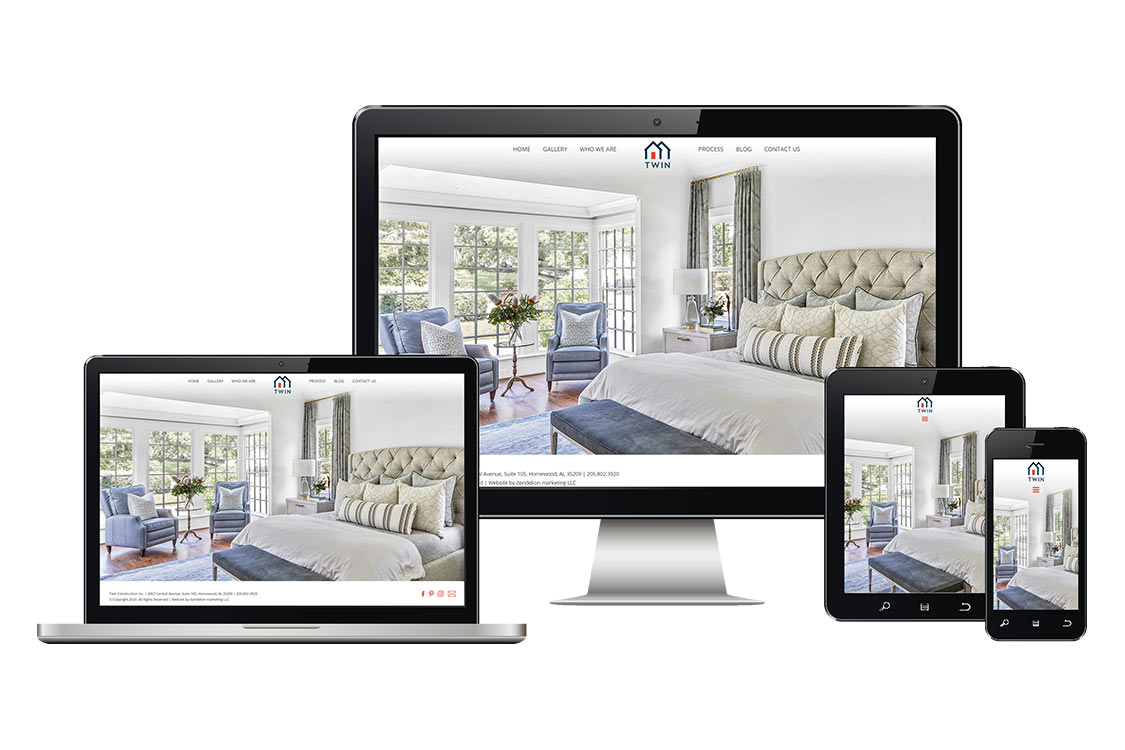The image features an array of various electronic devices displaying the same content. In the center, there is a freestanding PC typically found in home settings. To the left, there is a laptop, while on the right, there are two tablets. Each screen showcases an identical image of a bedroom interior, suggestive of a home interior design application or website. The bedroom features a neatly made bed with a front bench, an expansive outer window, and tasteful decor, creating a cozy and inviting ambiance. At the top of the display, there is the word "twin" accompanied by two home icons, implying it may be part of a section or category related to twin-sized rooms or beds. The displayed content across all devices embodies a beautiful and well-designed home decor interface.